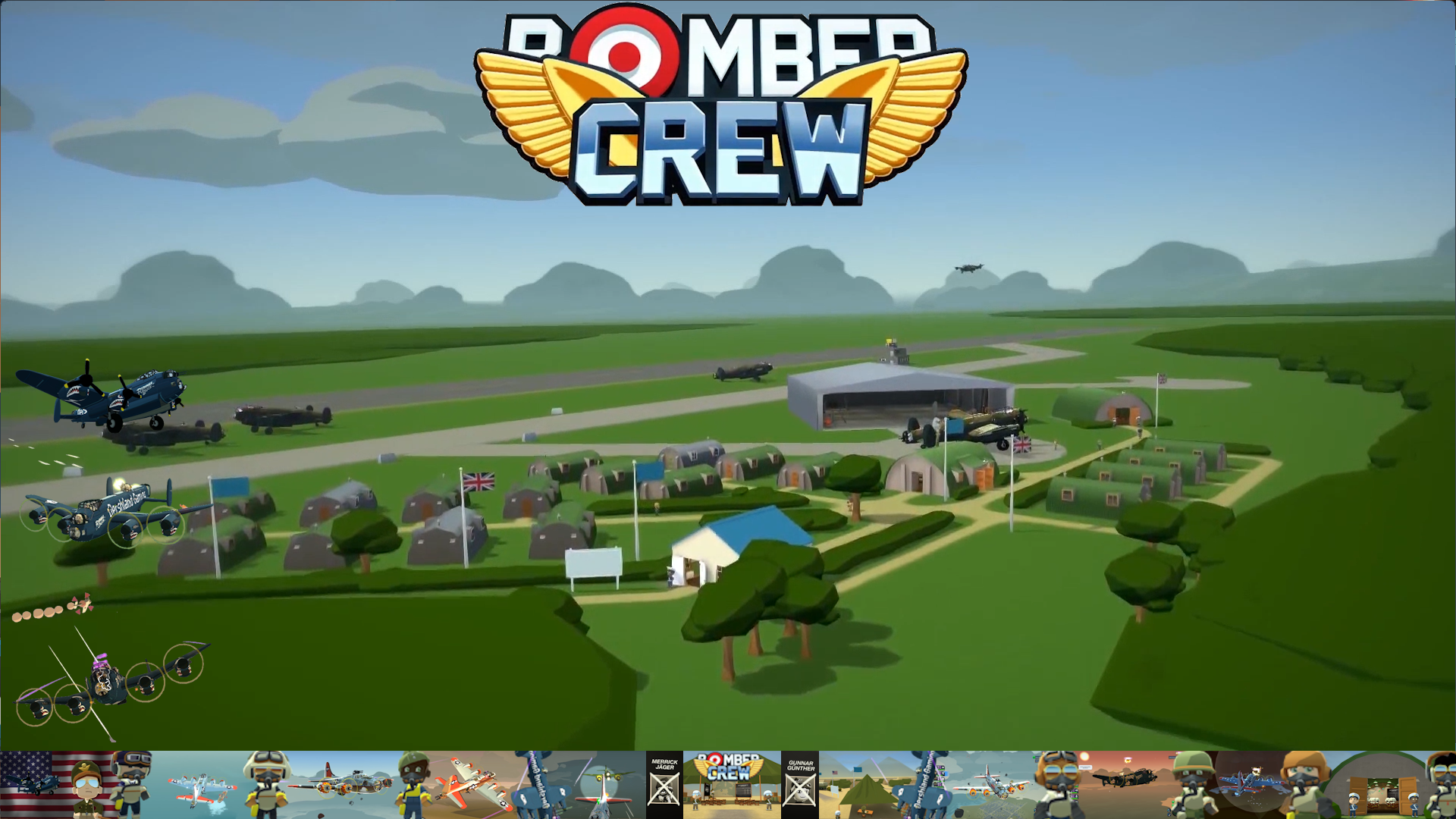This detailed digital rendering presents an air force base set against a backdrop of a blue sky with gray clouds. Central to the image, spanning from the middle to the left, are military barracks or a row of farmhouses, accompanied by an aircraft hangar slightly off-center to the right. Surrounding these structures are lush green grass and clusters of trees and bushes, particularly noticeable in the bottom corners. 

The base features multiple planes, including one positioned on the runway to the left, extending to the right, and others situated around the hangar—one in front and another behind. Additionally, an aircraft appears to be taking off from the runway, while another airplane hovers in the air near the clouds. These planes exhibit a vintage, World War II aesthetic, contributing to the historical military theme.

Highlighting the image is the text "Bomber Crew" at the top center, styled in white and blue with the letter 'O' resembling a red and white target symbol. Adding to the detail is a British flag flying at the military base. The overall setting resembles a scene from a strategy game app called Bomber Crew, viewed from a top-down perspective.